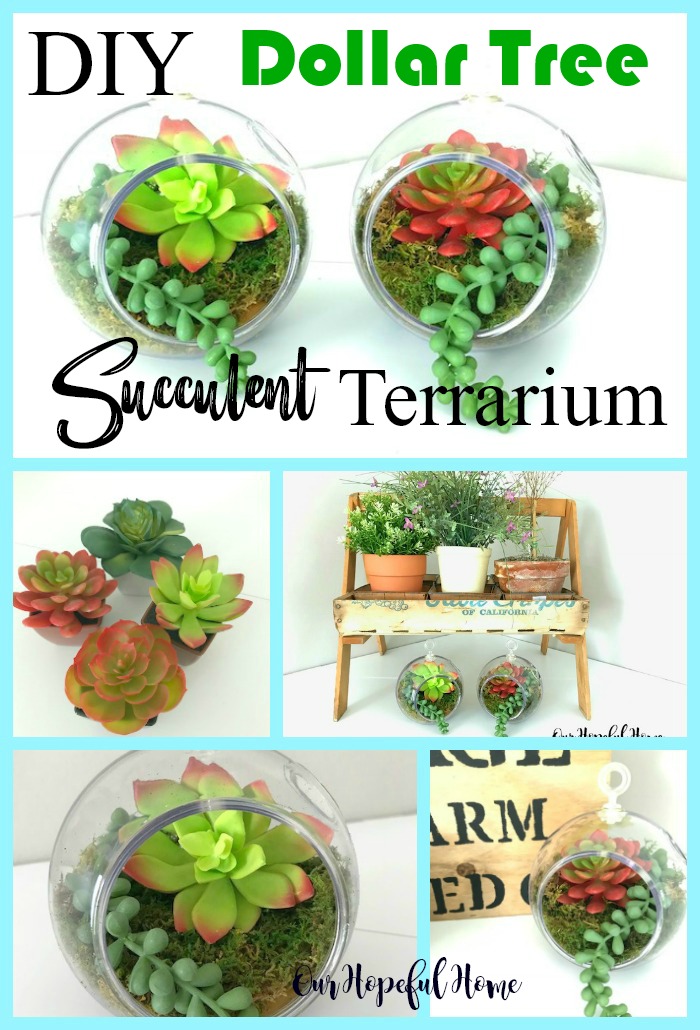This is a detailed advertisement for Dollar Tree labeled "DIY Dollar Tree Succulent Terrarium," showcasing a variety of do-it-yourself plant arrangements. The image exhibits five distinct sections with a white background and is bordered by a light blue trim.

At the top, there are two succulent terrariums in clear glass-like jars or cylinders, each containing vibrant succulents. One jar features a green succulent with dark red hues, and the other has a combination of deep red and green plants. These same terrariums also appear beneath a wooden bench, and again in the lower right quadrant of the image, reinforcing their presence and providing multiple views from different angles.

In the middle section, four colorful succulents are displayed in small containers, contributing to the lively visual appeal. On the right side, a wooden bench holds three additional plants, resting in various pots; some are brown, some white, and others are clear glass. Placed below the bench are the terrariums seen, connecting the different parts of the display.

The lower right quadrant features a green succulent reminiscent of jade, sitting on a platform with a partially visible sign behind it, displaying only a few legible letters, "A-R-E-D-R-M." Prominently, across the bottom of the image, there is text stating "Our Hopeful Home," tying the entire visual presentation together and enhancing the inviting, homemade aesthetic of the advertisement.